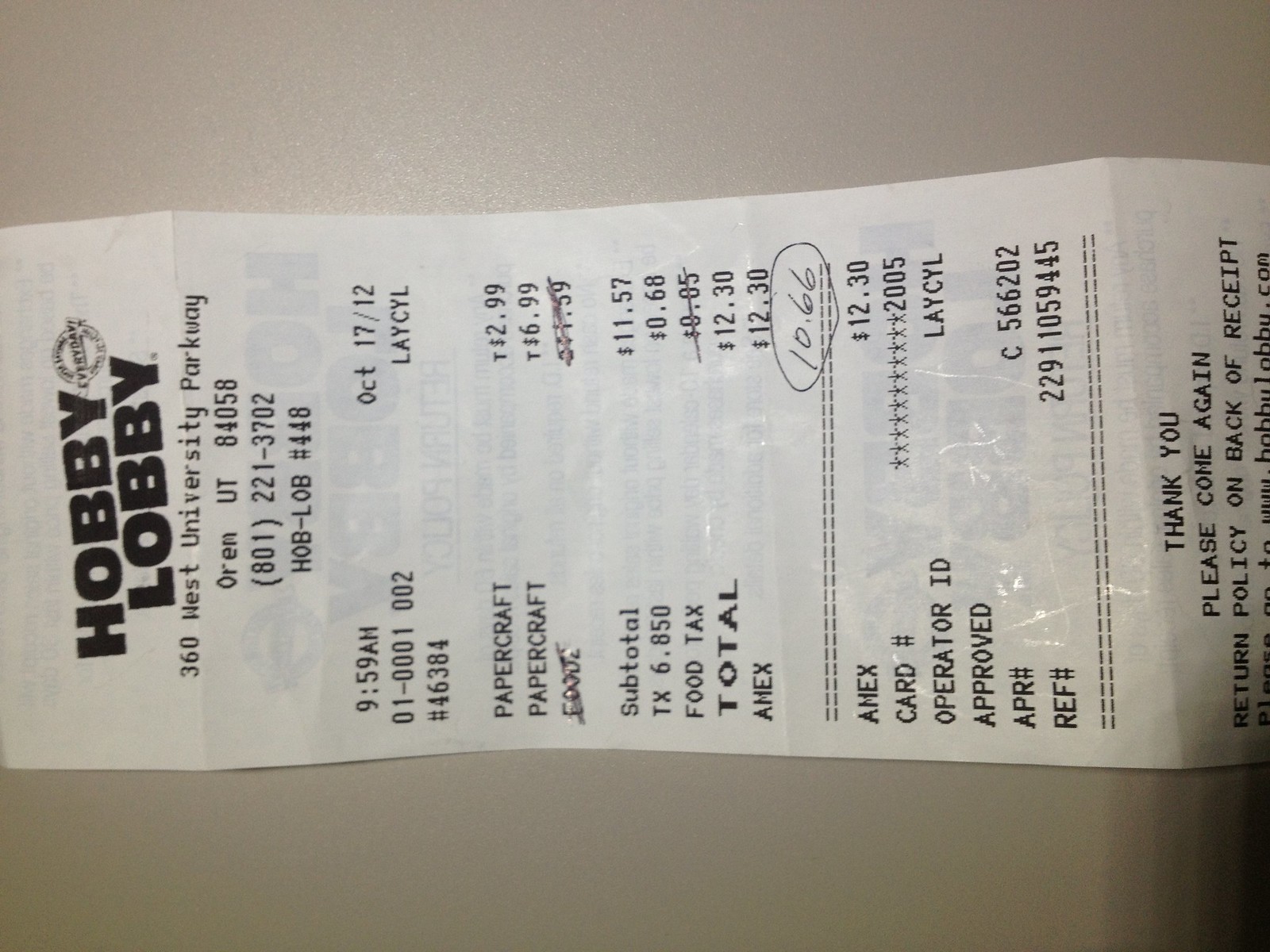The photograph captures a horizontally placed receipt from Hobby Lobby set against a light gray background, necessitating a sideways read due to its orientation. On the left-hand side of the image, "Hobby Lobby" is prominently displayed in dark, bold, black lettering. Below that, the store's address is detailed in smaller text: "360 West University Parkway, Orem, Utah 84058," followed by the contact number "801-221-3702." The receipt also includes a store identification, "HOBLOB #448."

The transaction details are visible beneath this header, marked by the date and time "October 17th at 9:58 a.m." The items purchased include two paper craft products priced at $2.99 and $6.99 respectively. An additional item, seemingly food, was initially listed and later crossed out along with its amount. The original subtotal was $11.57, with a tax of $0.68, bringing the total to $12.30 before adjustments.

Subsequently, the receipt was manually corrected, and the new total charged was $10.66. There's a note indicating payment made via American Express (Amex) with the original amount of $12.30 still legible. Additional details are present but not fully captured in this description.